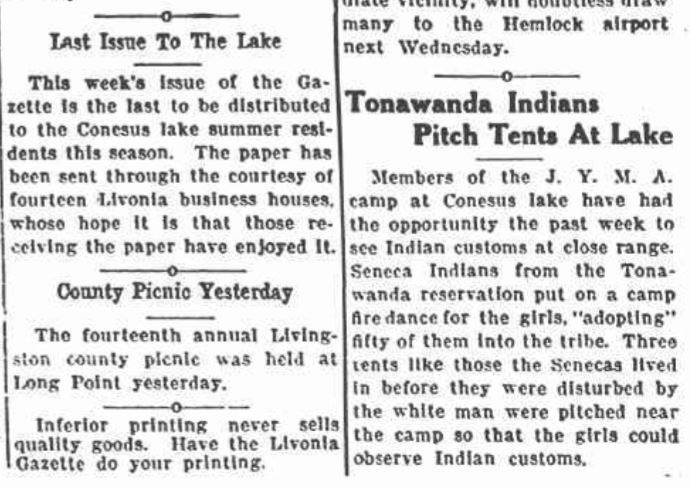This scan appears to be a section of a newspaper, likely from the right side of a larger article and adjoined by smaller advertisements or articles on the left. Set against a white background with black text, the main headline reads, "Last Issue to the Lake." Below it, the text announces that this week's issue of the Gazette is the last of the season to be distributed to the Knesset Lake summer residents. It explains that the paper has been generously sent out courtesy of 14 Livonia business houses, with a note of appreciation hoping that readers have enjoyed it.

Additional sections of the newspaper include a piece titled "County Picnic Yesterday," which reports on the 14th annual Livingston County Picnic held at Long Point. Another advertisement advises readers that "Inferior Printing Never Sells Quality Goods," promoting the Livonia Gazette's printing services. 

To the right, an intriguing article begins with the headline "Tonawanda Indians Pitch Tents at Lake." It describes how members of the JYMA camp at Knesset Lake had an educational encounter with Seneca Indians from the Tonawanda reservation. These visitors conducted a traditional campfire dance and adopted 50 girls into the tribe, setting up three traditional tents for the girls to observe Indian customs first-hand. 

The newspaper also contains scattered compression artifacts around the letters, likely due to the scan quality. Adjacent articles and advertisements provide a glimpse into the local events and services available to the community.